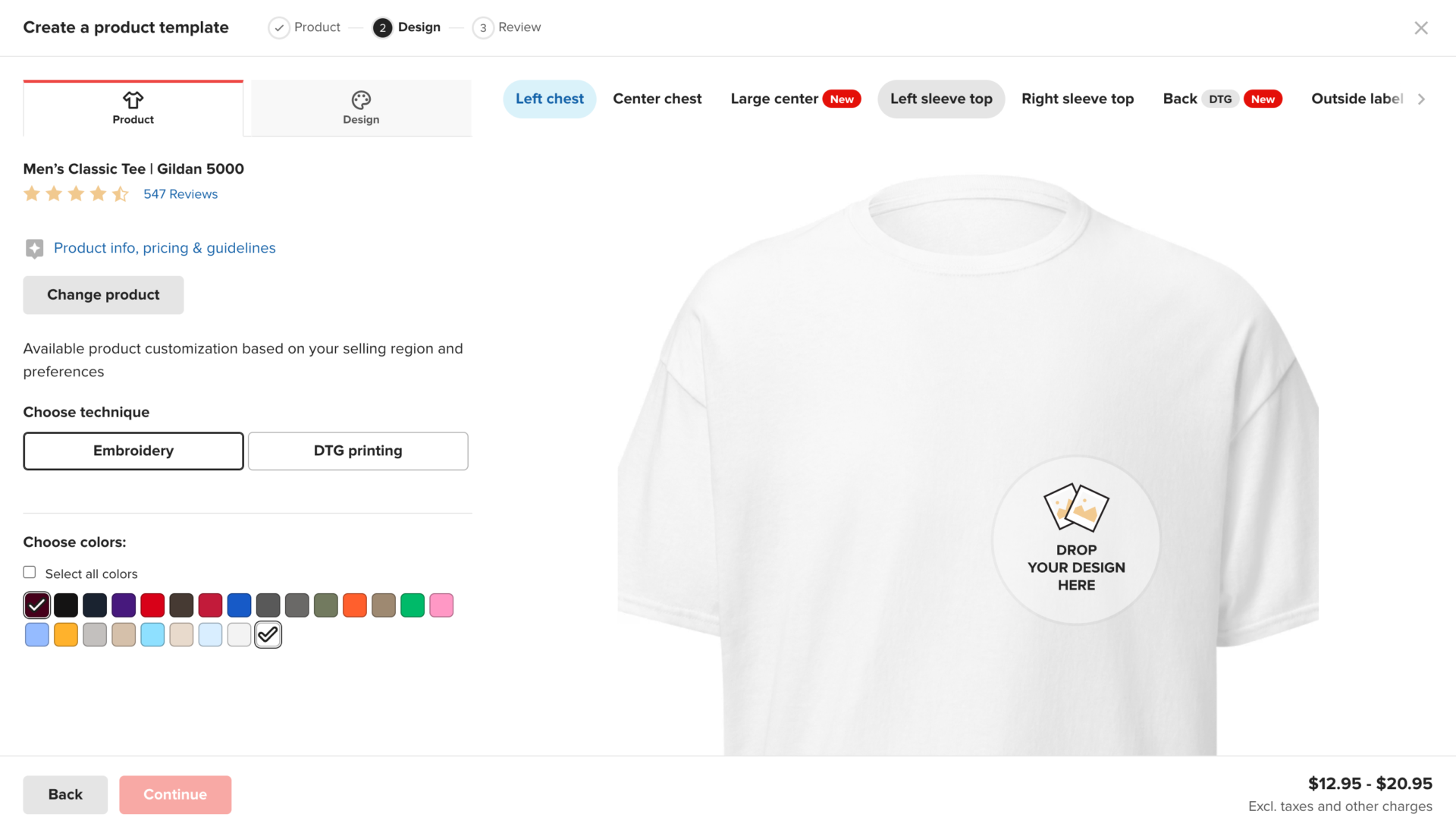**Detailed Product Customization Interface Description**

At the top left-hand corner of the interface, there is a title bar that reads "Create a Product Template." Below this, the interface is divided into three main sections labeled "Product," "Design," and "Preview." A red line demarcates the transition between these sections.

In the "Product" section, an image of a plain white T-shirt is displayed prominently, accompanied by the words "Men's Classic Tee, Gildan 5000." This product has a rating of 4.5 stars out of 5, based on 547 reviews, next to which are links for "Product Info," "Pricing," and "Guidelines." Above this item description is a button labeled "Change Product," followed by a note indicating that available product customizations are based on the user's selling region and preferences.

Adjacent to this, in the "Design" section, there is a puzzle piece icon labeled "Design." Below are multiple placement options for the design, including "Left Chest," "Center Chest," "Large Center," "Left Sleeve Top," "Right Sleeve Top," "Back, D16," and "Outside Label." Each area of the T-shirt that can be customized is labeled accordingly. At the center of the T-shirt image is a circle that says "Drop your design here," along with clip art of two images, indicating where users can upload their designs.

To the right of the design options, there are the customization settings. These settings start with a dropdown to "Choose Technique," displaying options like "Embroidery" and "DTG Printing." Below it, users are prompted to "Choose Colors," with a checkbox labeled "Select All Colors" (which is currently unchecked), followed by a palette of different color swatches.

At the bottom of the interface, there are navigation buttons labeled "Back" and "Continue," with the "Continue" button highlighted in red, encouraging users to proceed to the next step.

This comprehensive interface offers users a detailed and intuitive way to customize their product designs with ease.